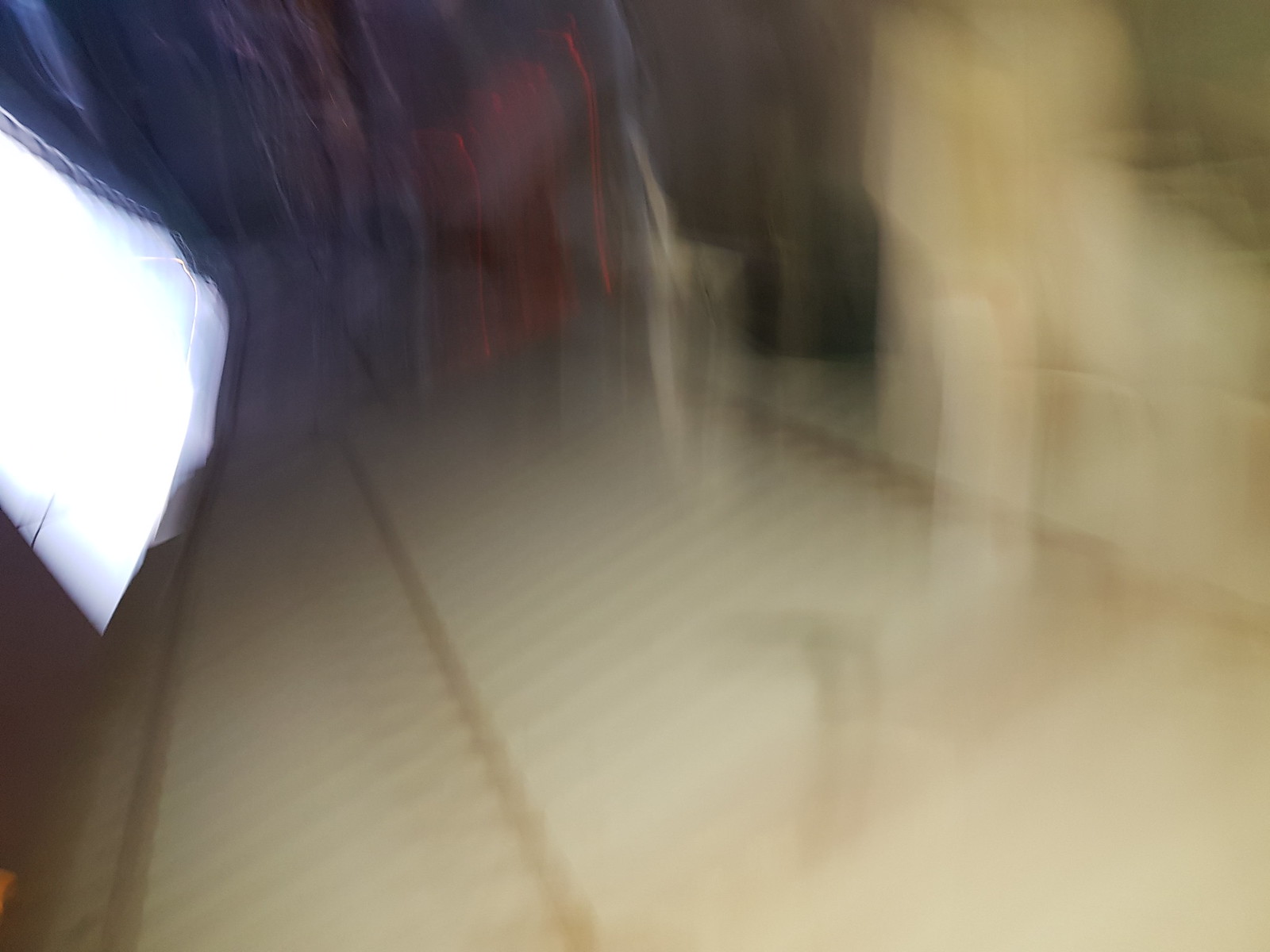This extremely blurry photograph appears to have been taken with a significant amount of motion blur, making it challenging to identify specific details. The image depicts a scene that resembles a sidewalk or walkway with beige or light-colored flooring, possibly featuring brown stripes. To the left, there is a bright white light source, which might be a light bulb or another form of illumination. In the center, the ground shows what could be interpreted as a wooden object, perhaps a laundry rack or a window shutter, positioned flat on the ground. There's a vague outline of people standing or walking on the sidewalk; one of them seems to be wearing a blue shirt and beige pants, while the other appears to be dressed entirely in white. Additionally, on the right side of the image, there's an indistinct white blob, which could possibly be a sofa or another large object. The overall impression is of a snapshot taken hastily, possibly in a subway station or a similar urban setting.